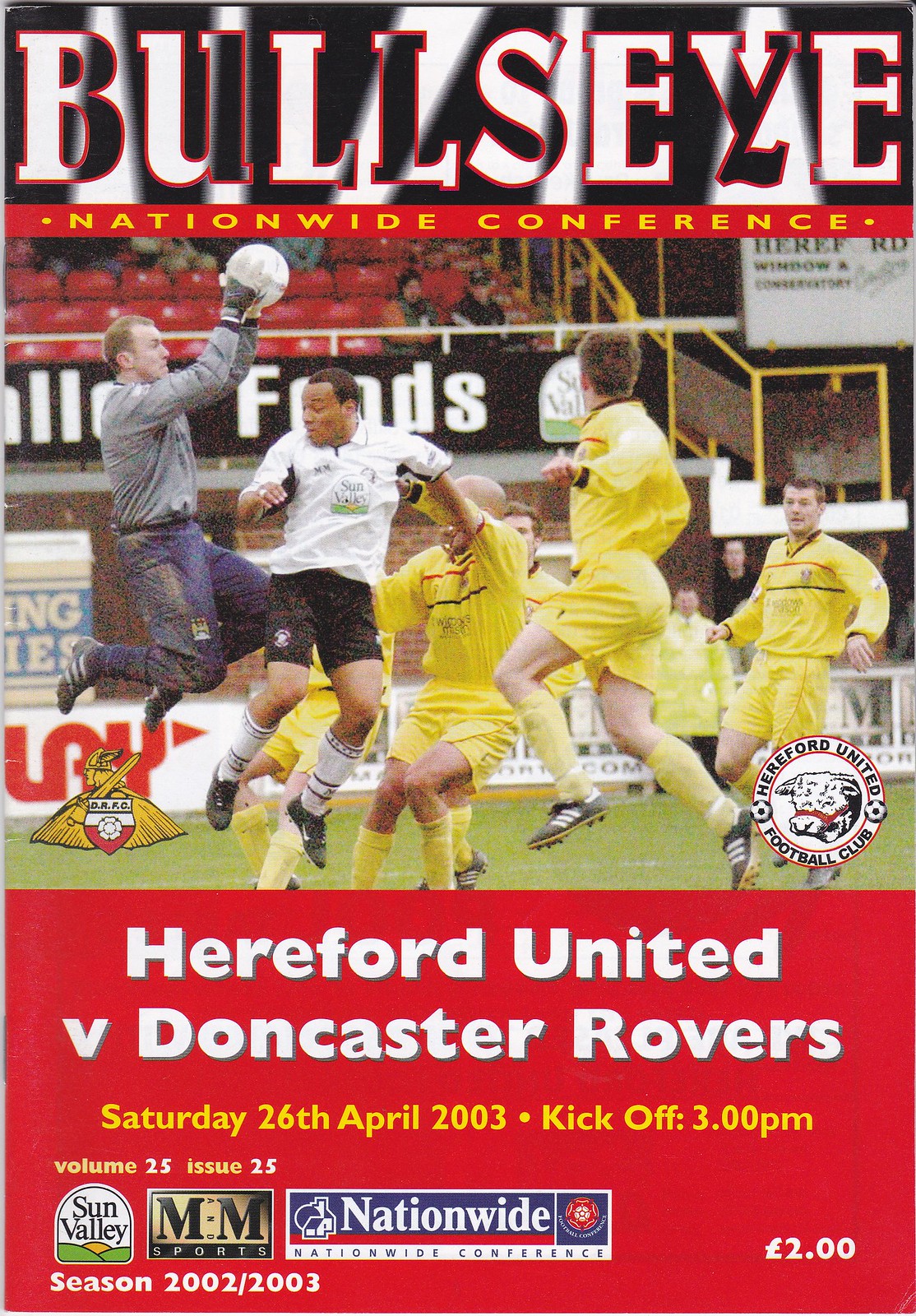The cover of Bullseye Magazine features a bold header reading "Bullseye" in striking white letters outlined in red with a black overlay. Below, it highlights the "Nationwide Conference" in vibrant red, with the text in yellow letters. Dominating the center, a dynamic photo captures men midair during a soccer match on a green playing field. One player, in a gray and blue outfit with gloves, is grasping a white ball. Another player in a white shirt and black shorts watches intently, while a third in an all-yellow jersey and shorts also leaps into action. Several other players in yellow are seen paused mid-motion. At the bottom, it reads "Hereford United vs. Doncaster Rovers" alongside the match details: "Saturday, April 26, kickoff at 3 p.m.", along with "Volume 25, Issue 25, Season 2002-2003". The cover also features logos for the Hereford United Football Club and BRFC, and is priced at 2 pounds.